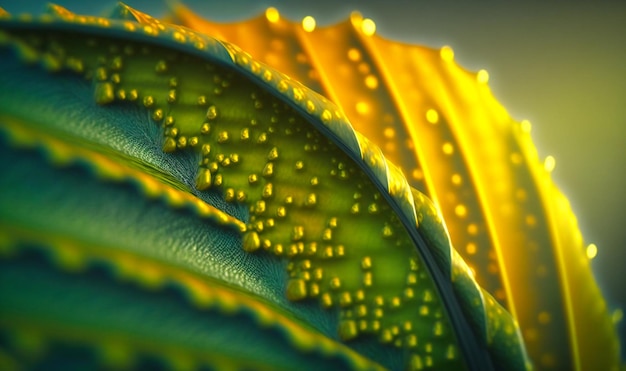This is an AI-generated close-up image of vibrant green leaves, emphasizing various shades of green and yellow, with subtle hints of blue. The leaves feature distinct rib-like lines and are oriented both to the left and right, creating a dynamic visual composition. Scattered across the surface are numerous small, round, shimmering objects that resemble either insect eggs, dew droplets, or tiny lights, adding an intriguing texture to the image. The backdrop is blurred, which accentuates the leaf details and the circular objects that range in color from light green to golden yellow. This digitally created image lacks additional objects or text, focusing purely on the detailed, slightly surreal depiction of the leaves.